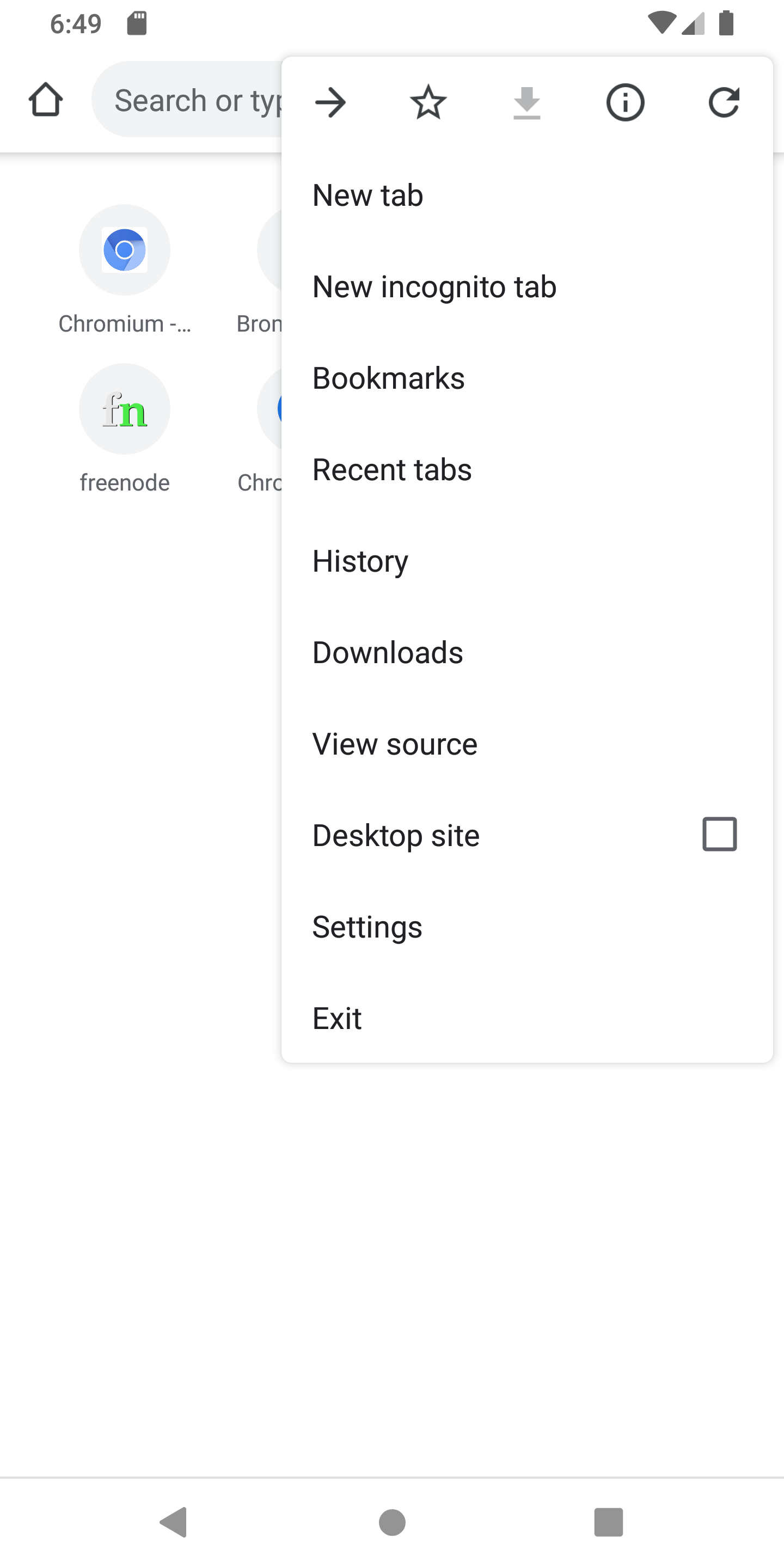Here is a detailed and cleaned-up description for the image caption:

---

The image captures a vertical screenshot, resembling the screen format of an Android or iPhone. At the very top of the screen, there are black letters displaying "649" accompanied by a memory card icon. In the upper right corner, typical status indicators are visible, including a Wi-Fi symbol showing two bars of signal strength and a fully charged battery icon.

Dominating the right side of the screenshot is a large white box, likely a drop-down menu or a settings panel. At the top of this box, there’s a series of symbols: a black arrow pointing to the right, a black-outlined star, a gray arrow pointing downward with a bar below it, a lowercase "i" enclosed in a circle, and a refresh symbol.

Below these icons, there are several tap-able options listed in black text:
- New tab
- New incognito tab
- Bookmarks
- Recent tabs
- History
- Downloads
- View source
- Desktop site (with a gray square and white interior to its far right)
- Settings
- Accent

Partially obscured by the white box, a search bar can be seen at the top, with the text "search or PYP" mostly cut off. Beneath this, a black-outlined arrow points upwards, followed by a partially visible gray bar.

Towards the upper right of the screen, opposite the white box, there is a gray circle with a white square inside and a pattern of blue circles in the middle. Below this, in black letters, is the word "cronium." Further down, another gray circle features faint gray lowercase letters "f" and "n" in grass green, with the text "free node" below it.

Two additional icons are almost entirely cut off by the white text box. What is visible includes partial gray circles: one marked with "B-R-O-N" and another with "C-H-R" (ending in "E" or "C") with some blue visible inside the circle.

At the very bottom, a faint gray line stretches horizontally across the screen. From left to right along this line are a play icon, a gray circle in the center, and a square icon.